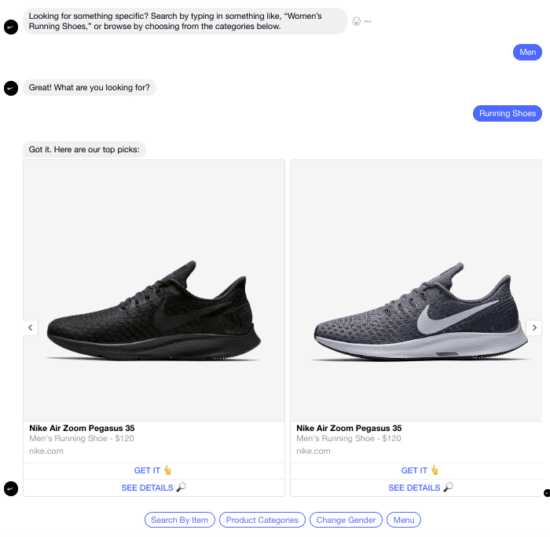The image depicts a chat interface designed for shoppers looking for shoes. The conversation begins with a user typing a specific query, such as "women's running shoes" or selecting from categories provided. The chat interface, possibly a chatbot, responds with a greeting and asks for more details. The user mentions they are looking for "running shoes." The chatbot acknowledges the request and presents two top picks: the "Nike Air Zoom Pegasus 35." Both shoes are priced at $120 and appear to differ only in color—one pair is all black, while the other is gray and white. The interface provides clickable buttons for "Get It" or "See Details." Additional options at the bottom include searching by item, browsing product categories, changing gender preferences, or accessing a menu. The chat system's exact nature—whether it involves a real person or an automated bot—remains unclear based on the image alone.